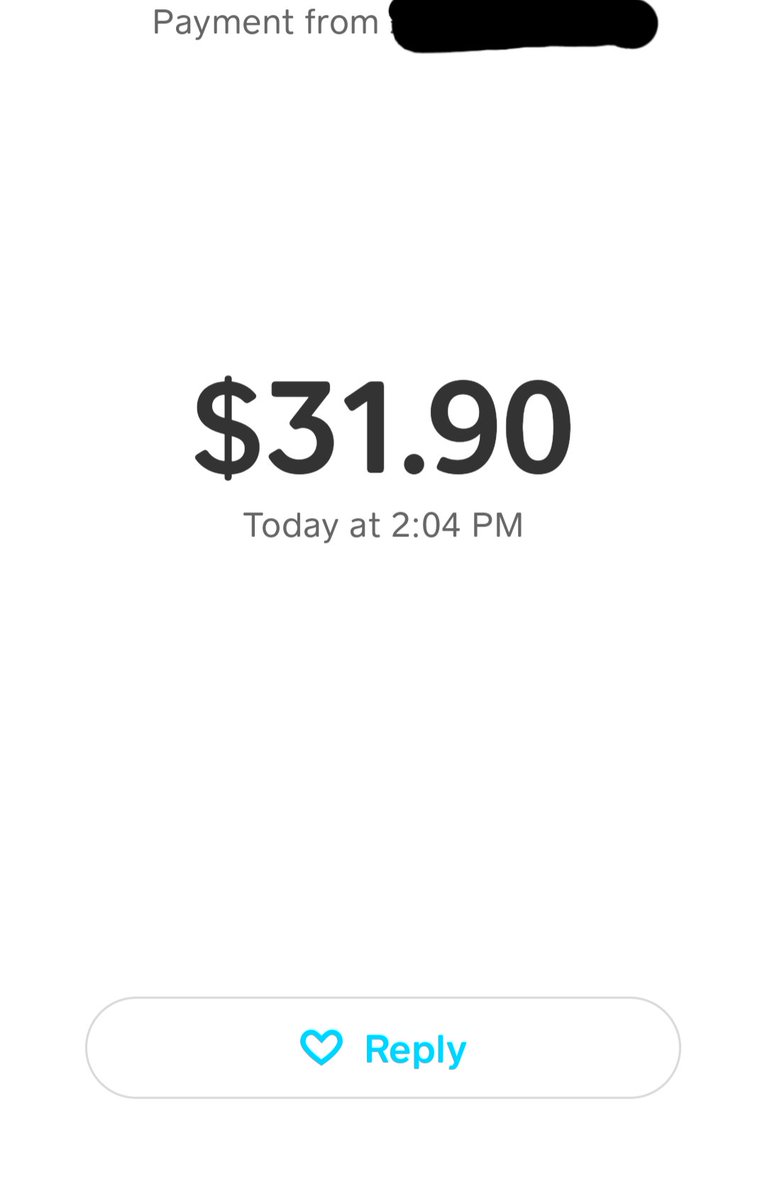The screenshot depicts a minimalistic white background. At the very top, in grey letters, it says "Payment from," followed by text that has been scribbled out with a black marker. In the center of the screen, bold black letters display the amount "$31.90." Directly beneath this, in smaller and lighter grey text, it reads "Today at 2:04 PM." At the very bottom of the screen is a white bubble outlined with a thin grey line. Inside the bubble, there is an empty teal heart icon next to the word "Reply" in teal. The screenshot is otherwise devoid of any additional elements or edges, blending seamlessly with the surrounding page.